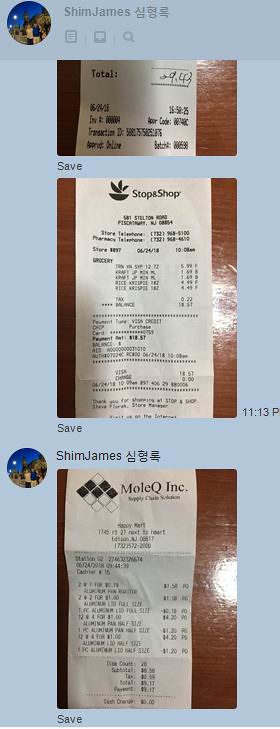The image is a screenshot of a messaging thread where a user named Shim James, identifiable by a circle icon and text in a foreign language next to his name, has sent three vertically stacked pictures of receipts. The photos, taken on a woodgrain table, show: 

1. A partially visible receipt at the top, with only the total amount of $9.43 or $9.49 clearly readable.
2. A full receipt beneath it from Stop & Shop, displaying item purchases and a timestamp of 11:13.
3. A folded receipt at the bottom from Mole Q Inc., entirely visible.

Each receipt snapshot includes a "save" prompt at the bottom.